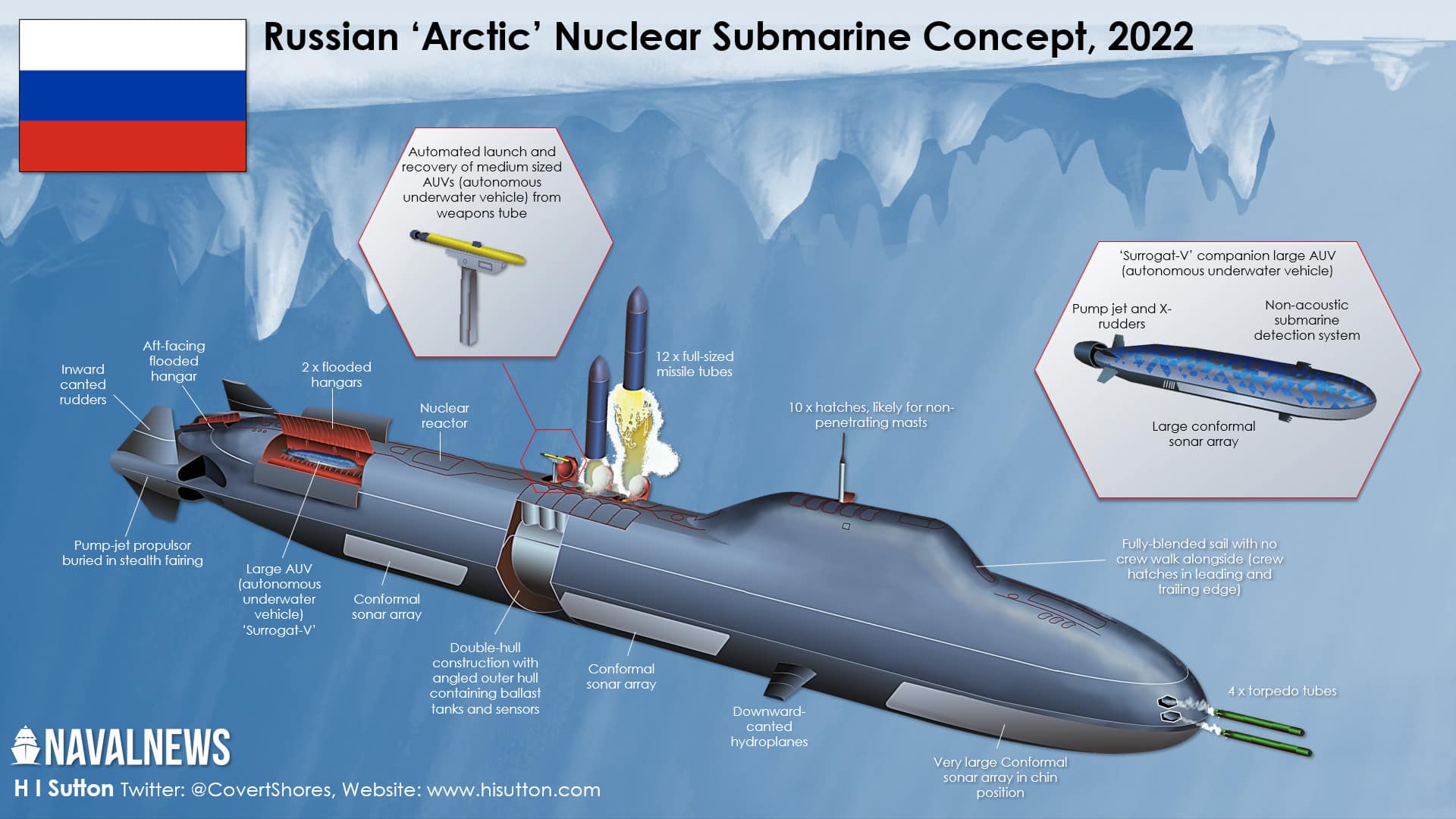The image is a detailed, informative drawing of a Russian Arctic nuclear submarine concept from 2022. The submarine, illustrated in an underwater scene beneath a glacier with sharp, jagged ice formations hanging down, showcases a variety of technical components and features. The main body of the submarine is blue with some red and yellow accents, particularly where rocket launchers might be situated. 

At the top left corner of the image, the text "Russian Arctic Nuclear Submarine Concept 2022" is displayed alongside a white, blue, and red Russian flag. The diagram is filled with numerous labels written in white, pointing to various parts and features of the submarine. These labels describe an array of advanced technologies and systems, including an "automated launch and recovery of medium-sized AUVs (Autonomous Underwater Vehicles)," "Surrogate V, Companion Lodge AUV," "pump jet and X-rotors," a "non-acoustic submarine detection system," and a "conformal sonar array."

The submarine has a complex design with a pump jet propulsor buried in a stealth fairing and a double hull construction featuring angled outer hulls that contain ballast tanks and sensors. It also includes two X-flooded hangers, a nuclear reactor, inlet canted rudders, downward canted hydroplanes, and a very large conformal sonar array. 

The bottom left corner of the image credits "Naval News HI Sutton," providing a Twitter handle "@CovertShores" and the website "www.hisutton.com." The intricate details and multiple hexagon-shaped insets within the diagram, including one showing a miniature submarine, further emphasize the technical sophistication of this submarine concept.